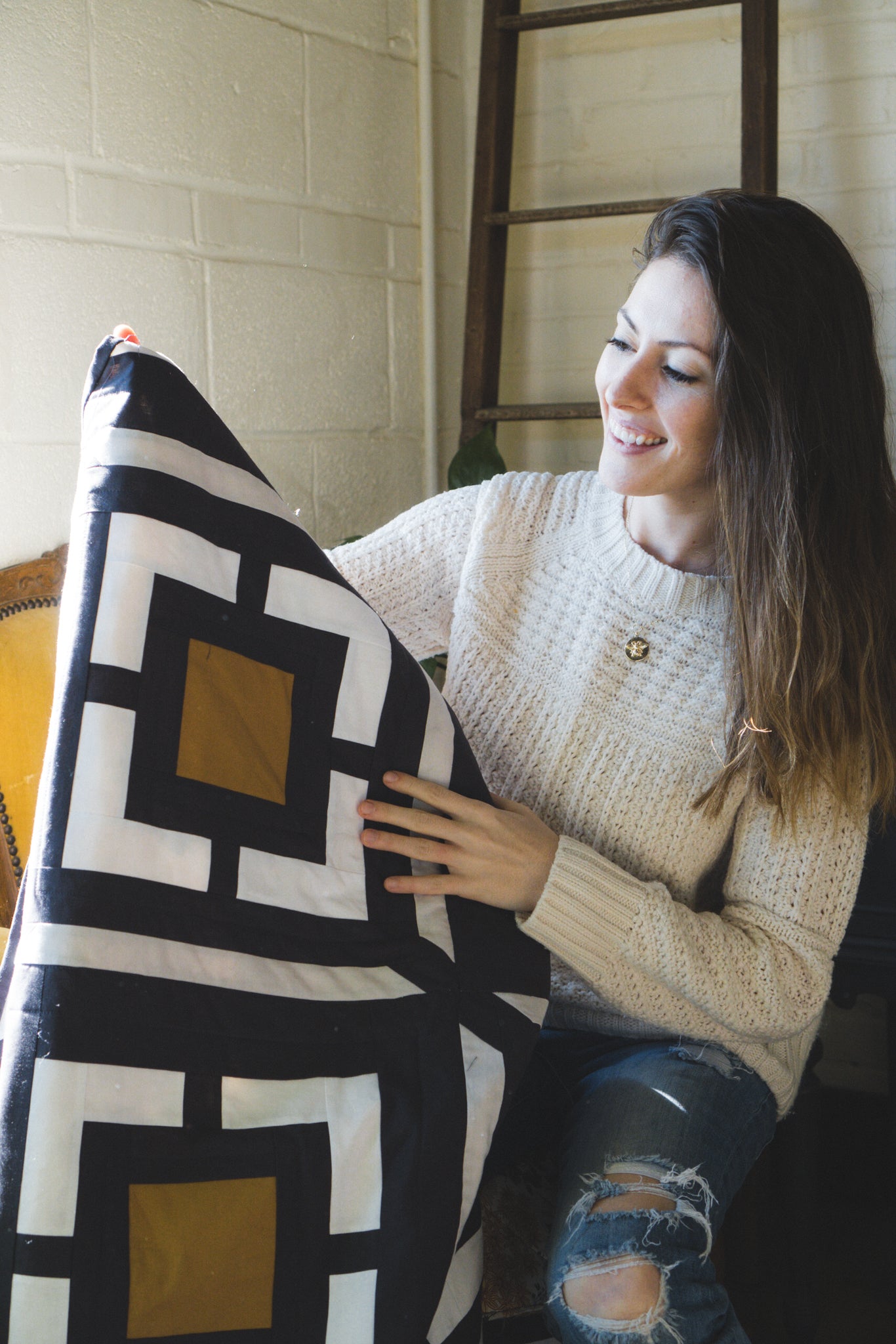In the image, a young woman, probably in her early 20s, sits on the right side of the frame with a radiant smile on her face. She has long brown hair and is dressed casually in a white cable-knitted sweater and blue jeans that are stylishly torn at the knees. She holds a beautifully patterned blanket, which is folded to show off its striking geometric design. The blanket features a dark blue background adorned with large brown squares outlined in white, reminiscent of a window pane. Her left hand is gracefully draped over the top of the blanket, as if she is either presenting it or admiring it. The backdrop includes a textured concrete-like brick wall and part of a wooden ladder leaning against it. A wooden object or frame is barely visible to the left of the blanket, adding a rustic charm to the setting. The woman's joyful expression suggests she might have just received the blanket as a thoughtful gift, adding to the warmth and happiness conveyed in the scene.